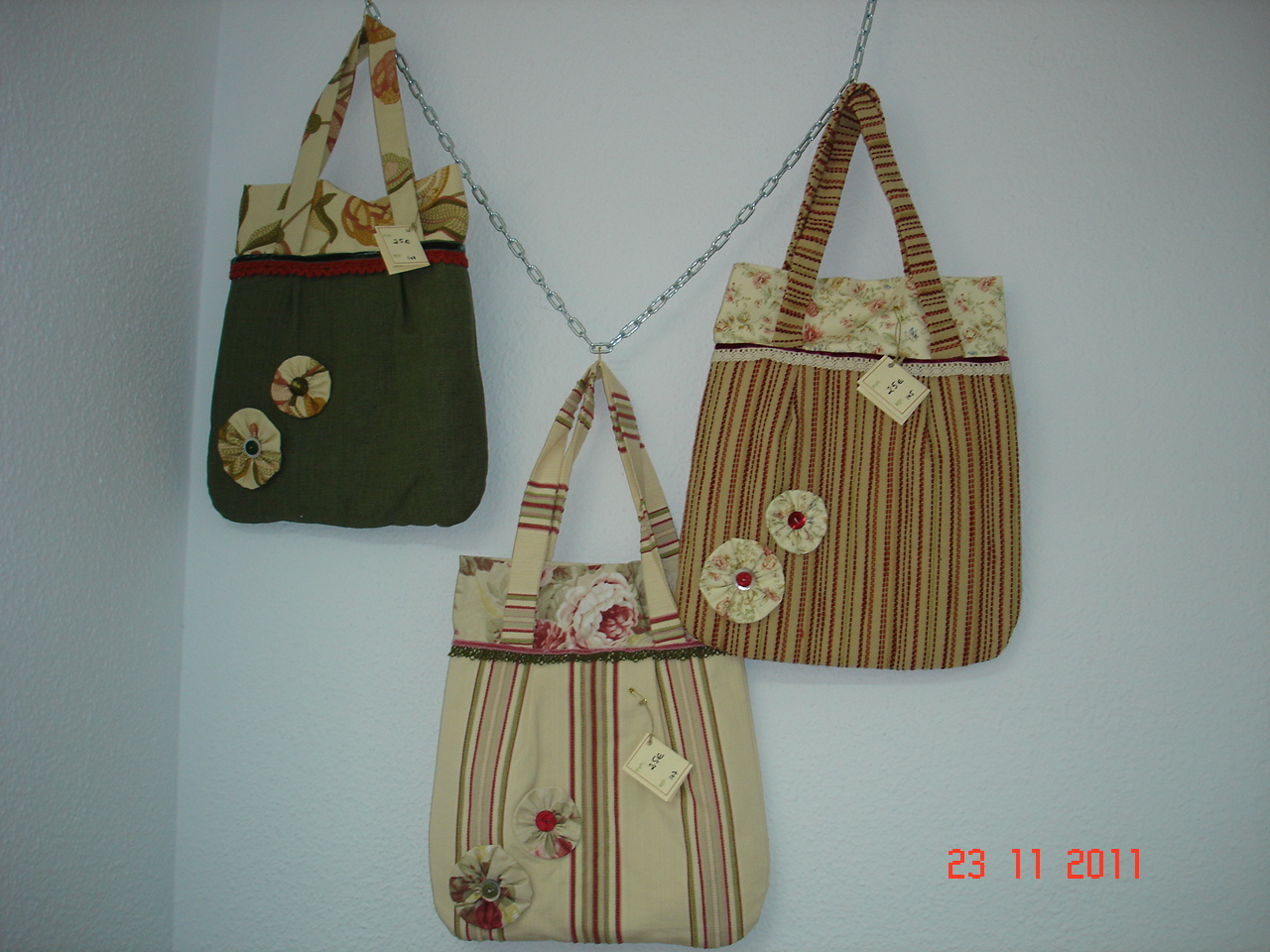The image shows three handbags hanging from a chain against a rough-textured, whitish-gray corner wall. The chain descends diagonally from the top left, forms a V-shape, and ascends diagonally to the top right. The handbags are positioned as follows: the first handbag is green with beige flower patterns and a gray handle with round patches, situated at the upper left. The second handbag, located at the peak of the chain's V-shape, is light tan with vertical red and greenish-gray stripes, and the handle features horizontal stripes. The third handbag, positioned to the upper right, is brown with vertical stripes and a lighter top adorned with flower designs. The image is timestamped 23-11-2011 in red at the bottom right corner.